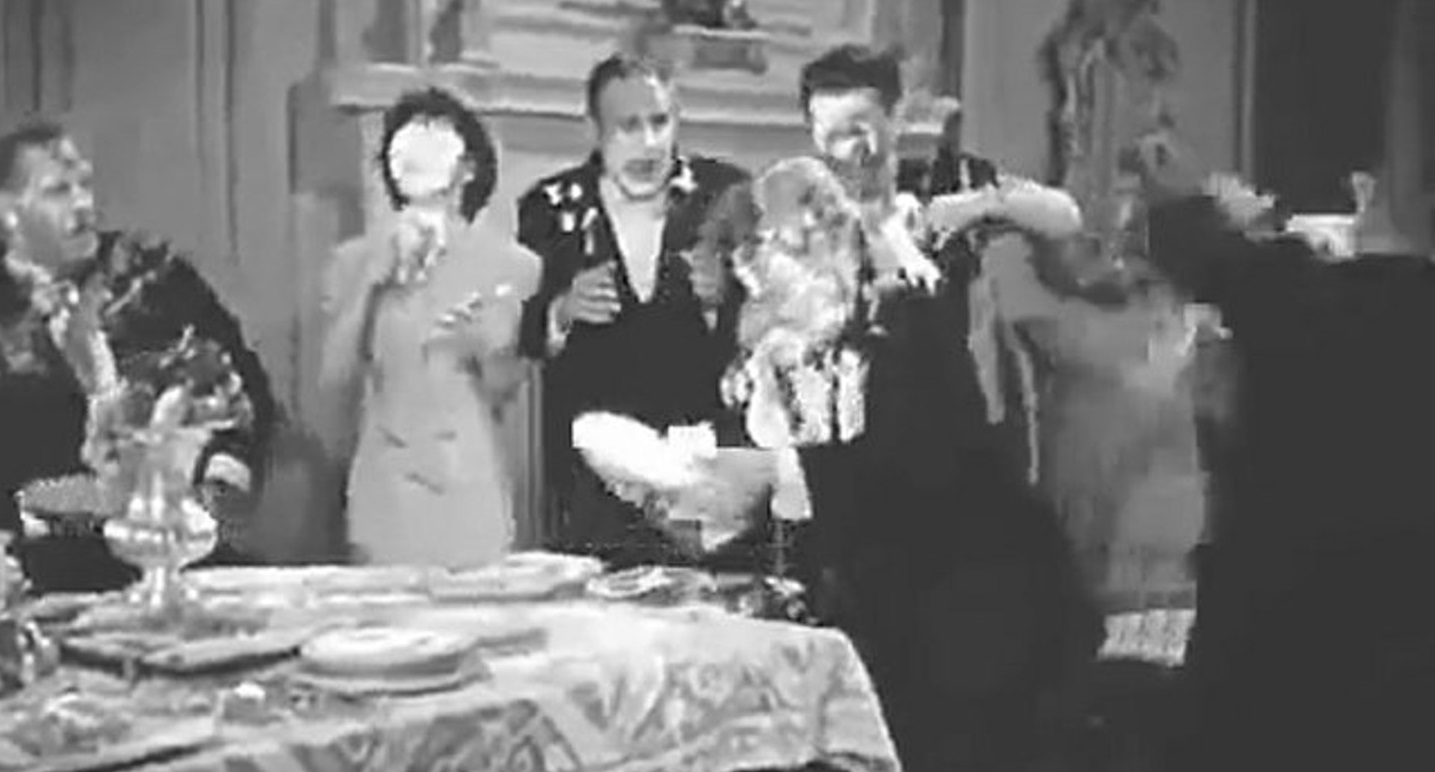In this somewhat blurry, black and white, landscape photograph, set likely in the 1940s or 1950s based on the fashion of the people involved, a chaotic and comedic scene unfolds. The setting is an expansive, ornate room, possibly reminiscent of a palace or a wealthy household, with a well-laid table featuring an urn-like centerpiece and elegant dishes. The image captures the aftermath of a lively pie fight among four men and two women, all attired in fine, albeit now disheveled, clothing. Pie remnants are splattered on their faces, clothes, and the lavish surroundings. One woman is entirely covered in pie, while another person, perhaps a man, is poised to throw another pie. The expressions range from shock to amusement, as even the gentleman at the center has a bit of pie on his face, epitomizing the jovial disruption of the formal setting. The image’s somewhat film-like quality, paired with the elaborate decor and the apparent spontaneity of the moment, suggests it might be a scene from a vintage movie.